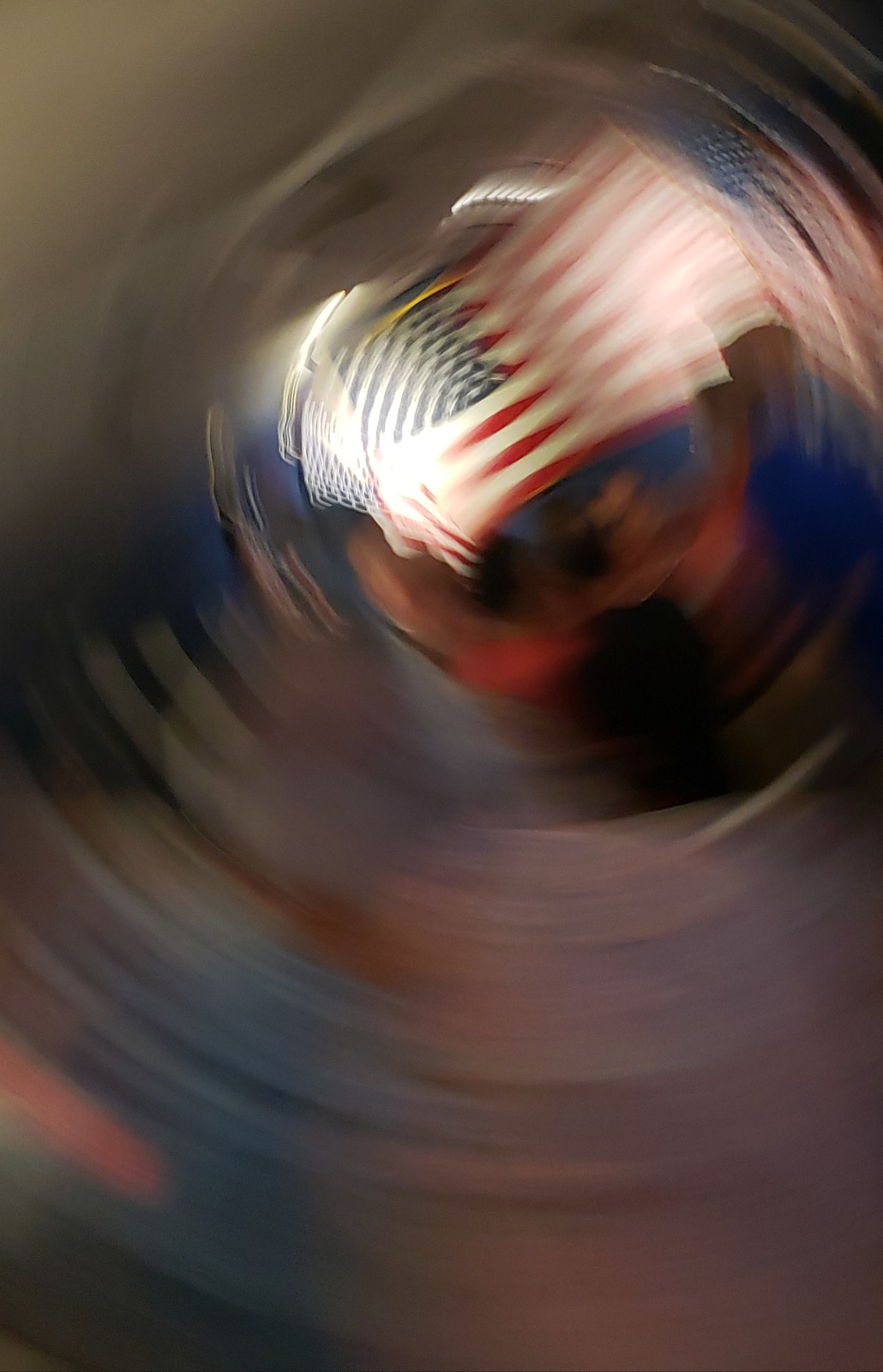This is a highly abstract and blurry color photograph with a vertically-oriented composition. The image features a mesmerizing, swirling pattern of light that forms a circular arrangement, capturing the viewer's attention. Positioned slightly above the center and towards the top right of the photograph is an American flag, which stands out distinctly despite the overall blurriness. Below the flag, there appear to be multiple figures, although their faces and details remain completely indiscernible due to the extreme lack of focus. The photograph is devoid of any text, visible individuals, animals, plants, buildings, motorized vehicles, or any kind of signage, fostering an enigmatic and ethereal visual experience.